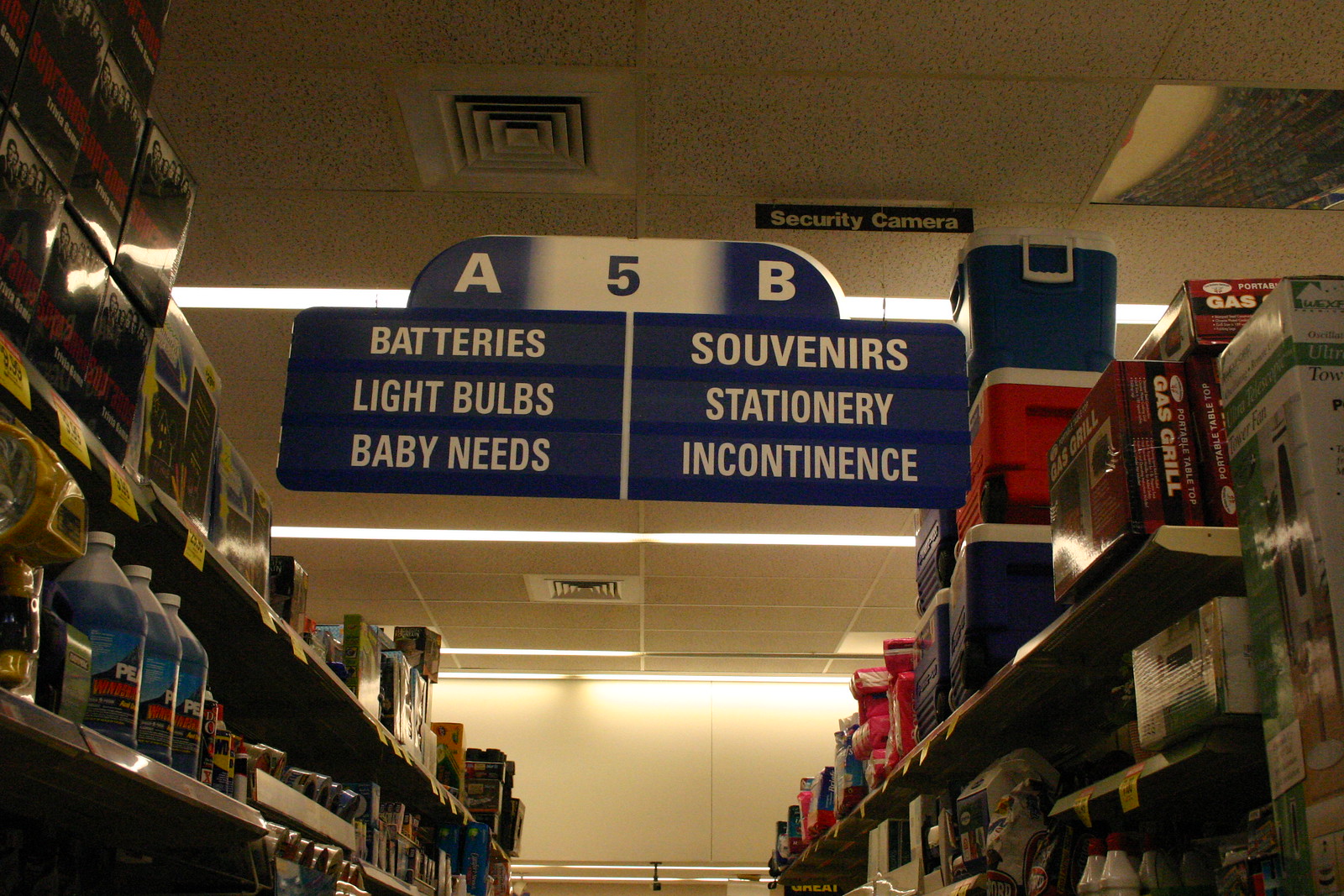Inside a large retail store—likely a grocery store or similar establishment like Target—the photograph captures a wide aisle scene from a slightly upward angle. On the left-hand side, a series of white shelves line the aisle, stocked with various cleaning supplies, including large jugs filled with blue liquid and sizable black boxes, although the specific contents of these boxes are difficult to discern.

On the right side, the top shelf is stacked with an assortment of blue and red coolers. Below them, colorful pinatas add a festive touch. Further down, a range of gas grills and other boxed appliances are neatly arranged along the bottom row of shelves.

A large, blue hanging sign dominates the upper section of the image, dividing the aisle into two clearly marked sections. The left section, labeled 'A,' directs shoppers to areas for batteries, light bulbs, and baby needs. The right section, labeled 'B,' points to souvenirs, stationery, and incontinence products. An aisle marker prominently indicating that this is aisle 5 adds a finishing detail to this busy retail scene.